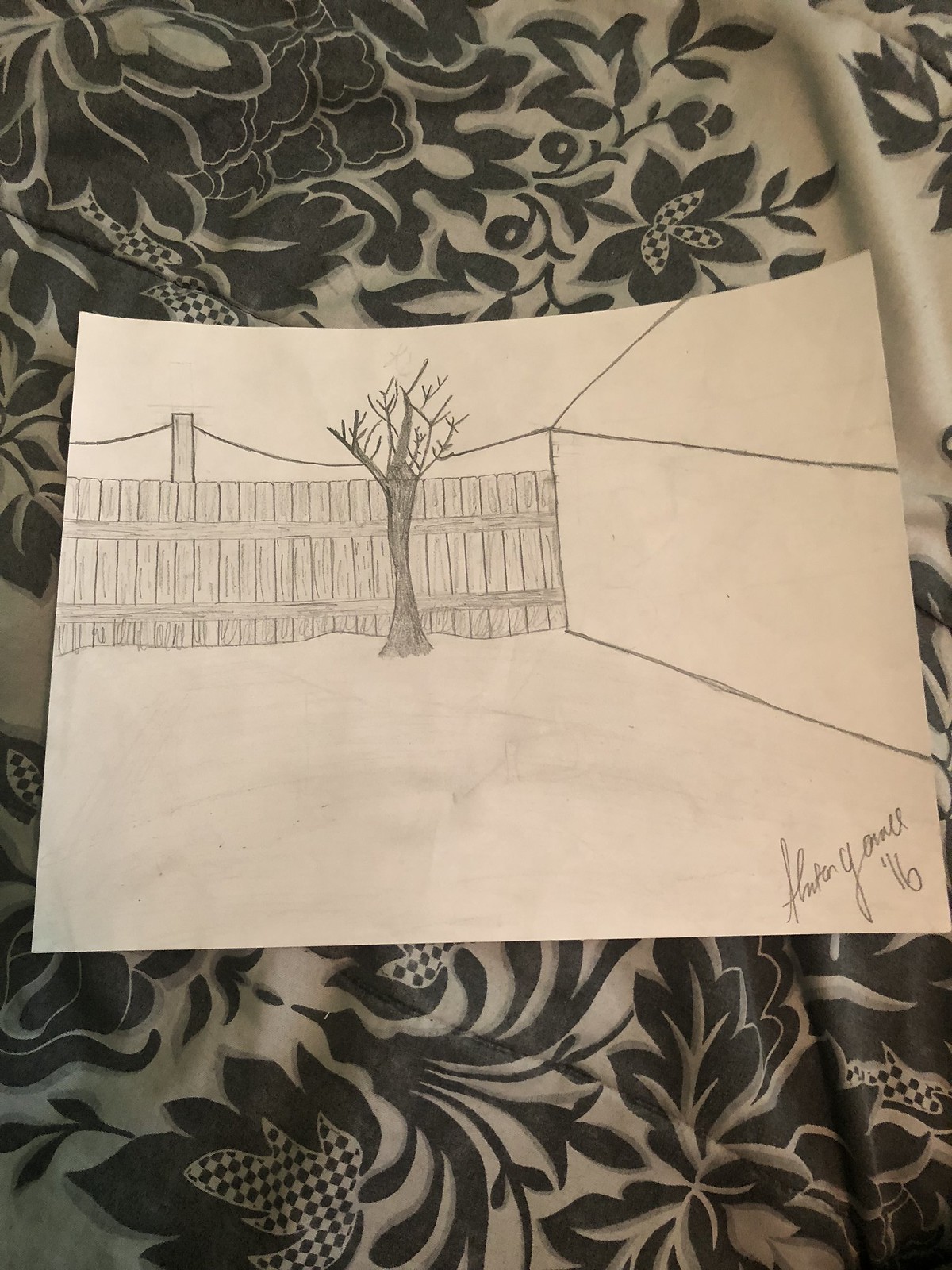The detailed pencil sketch rests on a piece of white paper, which has been carefully placed atop a crumpled, black and white floral cloth. This cloth background features intricate patterns resembling maple leaves and roses, adding a textured, monochromatic frame to the artwork. 

In the sketch itself, a wooden paneled fence dominates the scene, with vertical wooden planks forming the posts and longer horizontal planks connecting them. Positioned in front of the fence stands a dark, barren tree, rendered with darker pencil strokes that contrast sharply against the lighter fence. This leafless tree, stark and solitary, reaches slightly above the fence, adding a sense of height and depth to the composition. 

Behind the fence, a pillar with a rope hanging from either side suggests a washing line, subtly hinting at domestic life beyond the immediate scene. In the bottom right corner of the sketch, a barely legible signature accompanied by "'16" indicates that the drawing was created in 2016. 

This visually striking pencil illustration captures a quiet, evocative moment, framed by the elegant yet contrasting backdrop of a floral-patterned cloth.